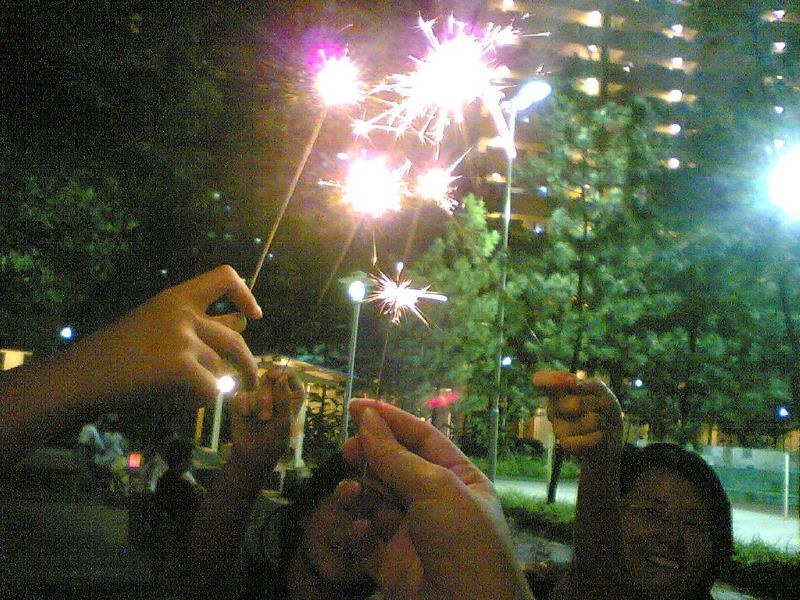In the nighttime photograph, a group of people are gathered outdoors, possibly in a park or courtyard, celebrating with sparklers in their hands. The background features tall green trees and a well-lit building, likely an apartment complex, illuminated on every floor. On the right side of the image, a bright city streetlight adds to the ambient lighting. Among the celebrants, two faces are visible: a blurry image of a small child and a smiling woman wearing glasses. This woman is holding up a brown stick that appears to be an unlit sparkler. Meanwhile, four other hands are raised, grasping lit sparklers that shine brightly with a tinge of purple at the edges. Behind the group, a couple can be seen holding hands or hugging, adding to the festive atmosphere.